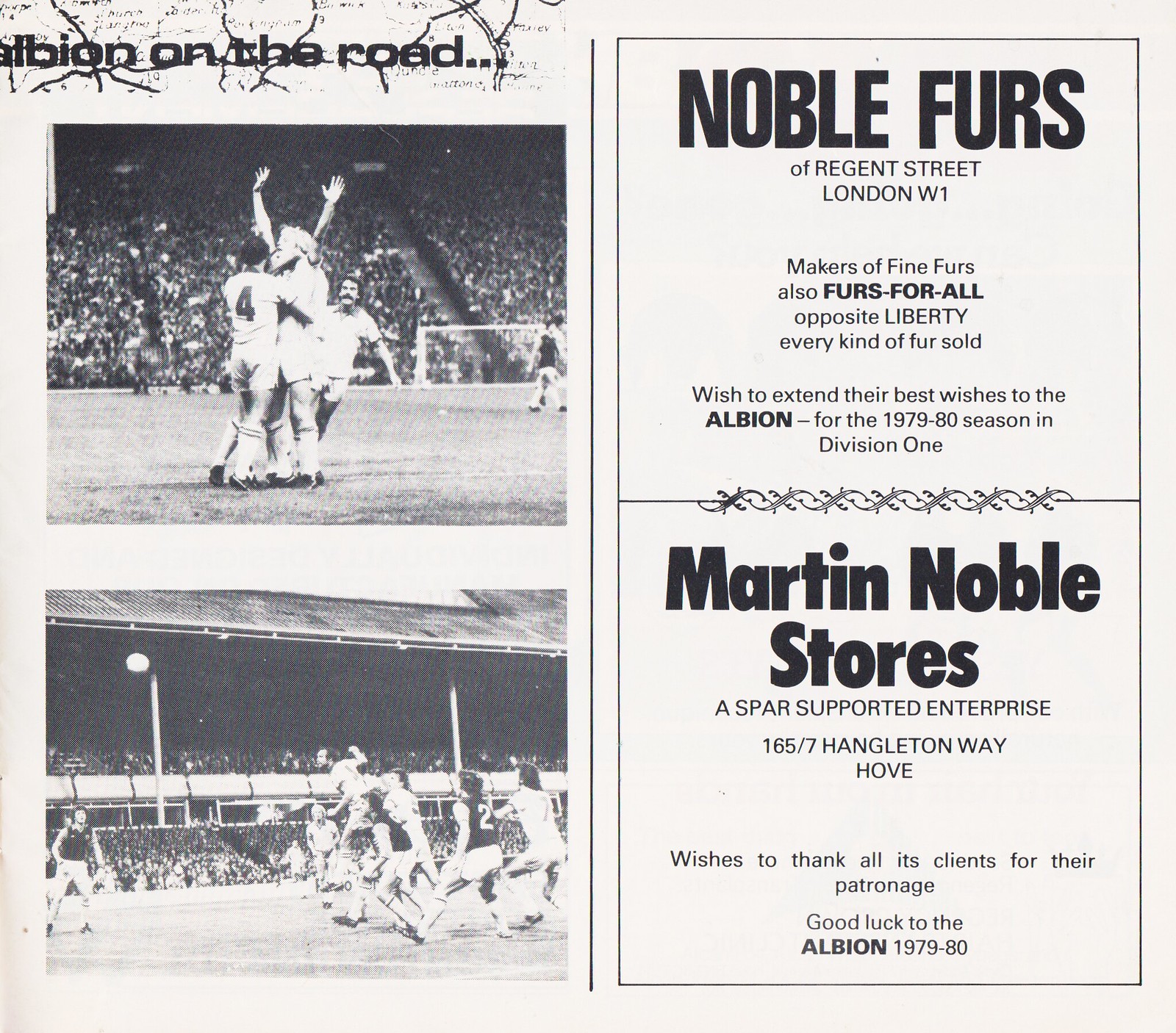This image, likely taken from an old newspaper or magazine, features a split layout with a light gray background divided by a thin black vertical stripe. To the left, the heading "Albion on the road..." is prominently displayed in bold black print, followed by two stacked black and white photographs. The top photo captures a celebratory moment on a soccer field: a player with arms raised in a V-shape is being hugged by a teammate in a white jersey numbered four. The bottom photo shows a mid-game scene, with players watching a ball high in the air, possibly following a header. The stadium and fencing are visible in the background.

On the right side, a tall rectangle with a black outline contains an advertisement split by a horizontal line adorned with curled ivy. The top half reads "Noble Furs of Regent Street, London, W1" and "makers of fine furs, also FURS-FOR-ALL opposite Liberty, every kind of fur sold. We wish to extend our best to the Albion for the 1979-80 season in Division 1." The lower half mentions "Martin Noble Stores, a SPAR-supported enterprise, 165-7 Hangleton Way, Hove," and expresses gratitude to clients along with good luck wishes to Albion for the 1979-80 season. The overall aesthetic, containing both the photos and detailed advertisement, supports the football team neatly within this nostalgic black and white layout.